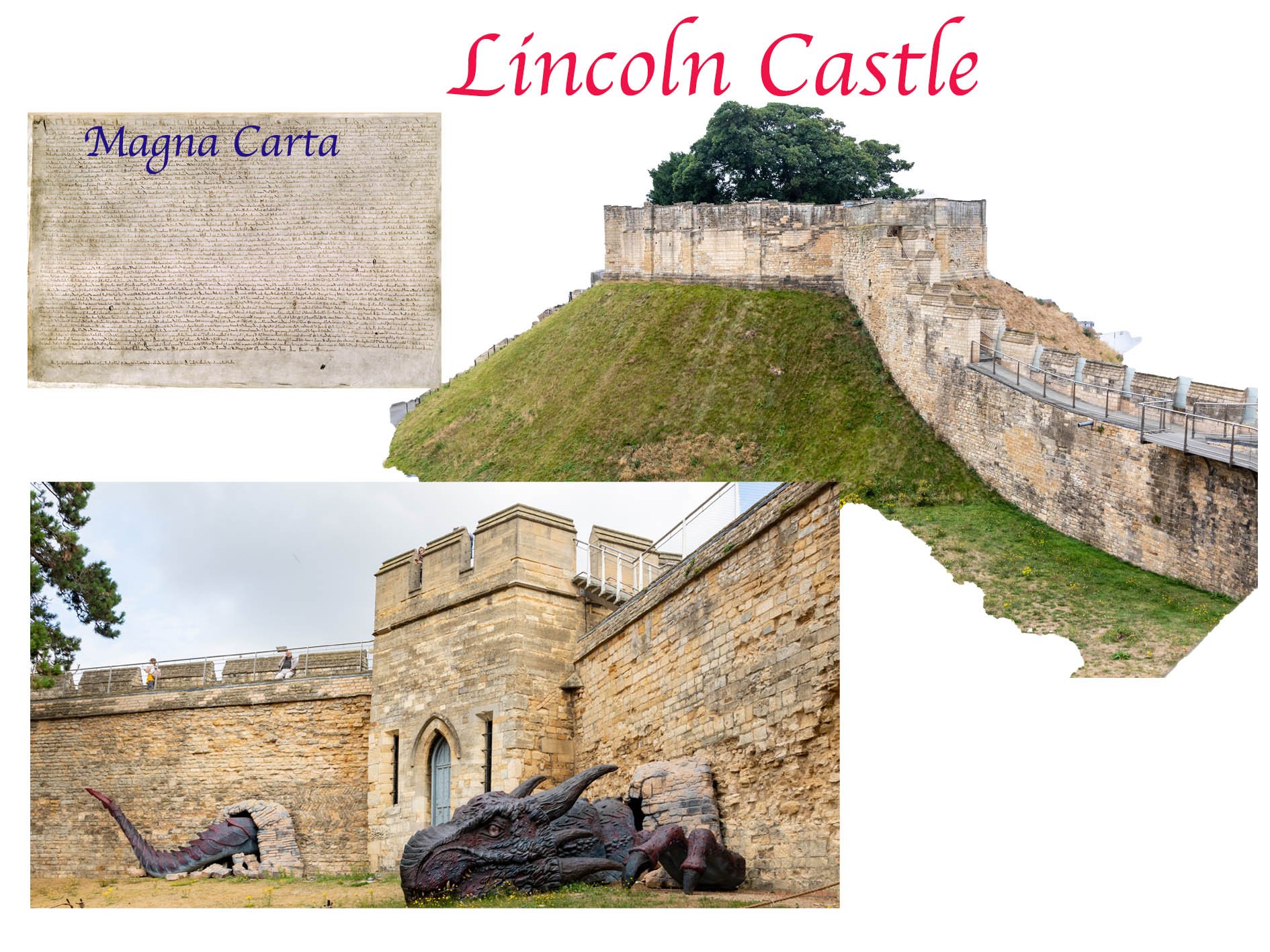The image features a weathered Lincoln Castle with its aged, light brown and cream brick walls, some of which are worn and eroded. Atop the castle wall, an oak tree prominently stands, adding a natural element to the historic structure that appears to be almost built into the hillside. In vivid red, italicized letters, "Lincoln Castle" is displayed at the top of the image, while at the top left, the words "Magna Carta" are written in blue on an older-looking document. At the bottom of the image, a fantastical blackish-red dragon seems to break through the castle wall, with its tail protruding from one side and its head and front claws emerging from the other, adding a mythical touch to the composition. The scene includes a bridge structure resembling the Great Wall of China, indicative of a graphic design project with transparent background areas and various cutout elements.